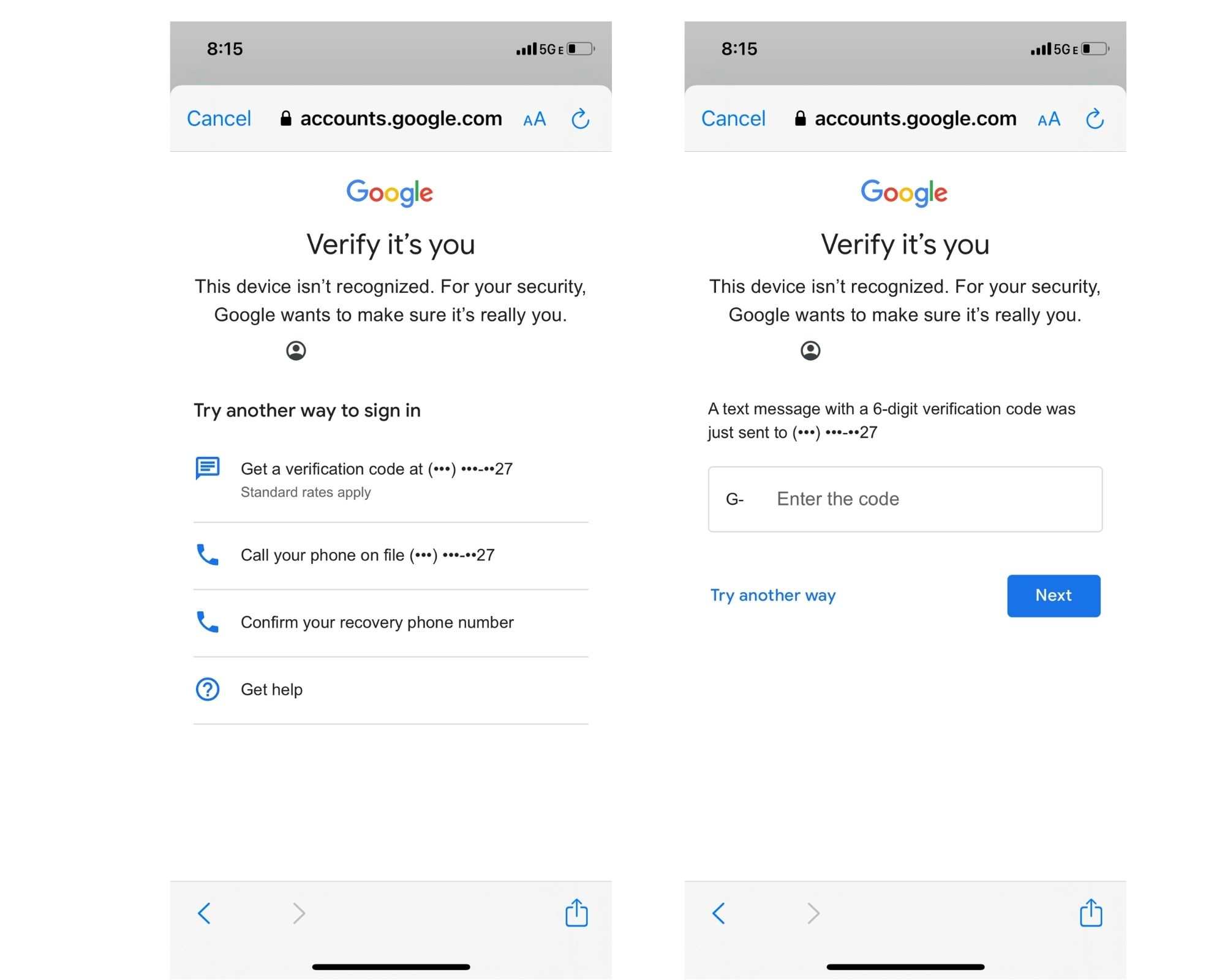The image features two distinct but analogous screenshots of a smartphone display, presumably on a verification page. Both screenshots display a gray status bar at the top, indicating the current time, network connectivity, and battery level of the phone.

Beneath the status bar, each image includes a light gray header containing various interface elements. On the far left, there is a blue "Cancel" link. Centrally, a black padlock icon is displayed next to the URL "accounts.google.com," reinforcing the security and legitimacy of the site. To the right, there is a small capital 'A' followed by a large capital 'A,' signifying text size options, and a blue refresh button depicted as a circular arrow.

Dominating the next section below the header, the prominent Google logo appears, with its letters "G-O-O-G-L-E" rendered in Google's signature multicolored scheme. Following the logo, a large text prompt states, "Verify it's you."

This is where the two images diverge: The left image shows additional prompts offering alternative sign-in methods, presenting several verification options for the user to choose from. Conversely, the right image has a straightforward prompt instructing the user to proceed by entering a six-digit verification code.

Overall, the visuals effectively communicate two different paths the user might encounter during the Google account verification process.